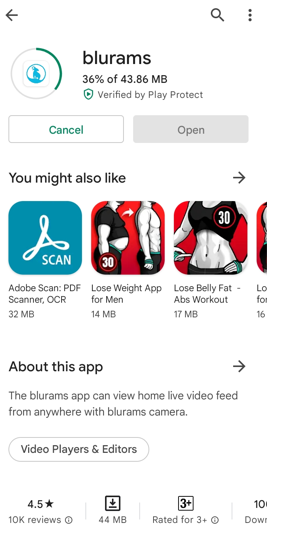This vertical mobile screenshot displays the download progress of the Blurams app on a white background. In the top left corner, there is a gray left-facing arrow. The main focus is the download status of the Blurams app, which is currently at 36% of the total 43.86 megabytes. The app icon, depicted as a gray outline circle with a blue logo in the center, features a green progress indicator on the right side showing the portion already downloaded. 

Below the progress indicator, "Verified by Play Protect" assures the app's safety. Further down, there are "Cancel" and "Open" buttons, giving the user control over the download process. The screen also displays suggestions under the heading "You Might Also Like," which includes apps like Adobe Scan, Lose Weight App, and Lose Belly Fat Abs Workout App, each accompanied by a right arrow for additional options.

Additional information about the Blurams app is provided under a section labeled "About This App," also with a right arrow. It mentions that the app allows users to view home live video feeds from anywhere using the Blurams Camera and classifies it under "Video Players and Editors." 

Towards the bottom, crucial app details are listed: the app has a 4.5-star rating based on 10,000 reviews, the download size is 44 megabytes, and it is rated suitable for users aged 3 and over. The number of downloads, although partially cut off in the lower right corner, indicates the app's popularity among users.